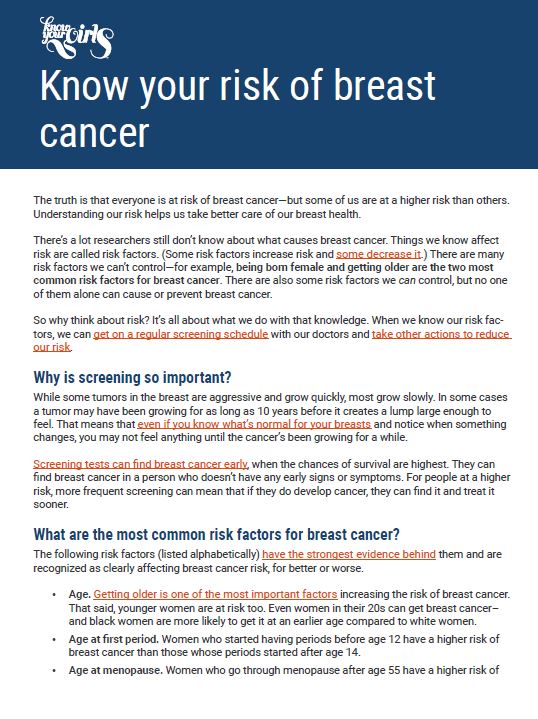The image features an informational screen divided into three distinct sections against a dark blue background. At the top, a cursive white logo with lined elements is prominently displayed. Directly beneath the logo, the text "Know Your Risk of Breast Cancer" is written in white. 

The first section of the screen, positioned right below the introductory text, contains three concise paragraphs. The primary text is in small black font, with certain key phrases highlighted in red and underlined for emphasis.

Following this is the second section titled "Why is Screening So Important?" This section also consists of predominantly small black text, interspersed with two segments of underlined red text to draw attention to critical points.

The final section, labeled "What Are the Most Common Risk Factors for Breast Cancer?", includes one comprehensive sentence followed by three bullet points. The first bullet point features some underlined red text. Unlike the upper parts of the screen, this section has a white background, adding contrast to the overall design.

Each segment is meticulously organized to present important information clearly, utilizing color and formatting to highlight key details.